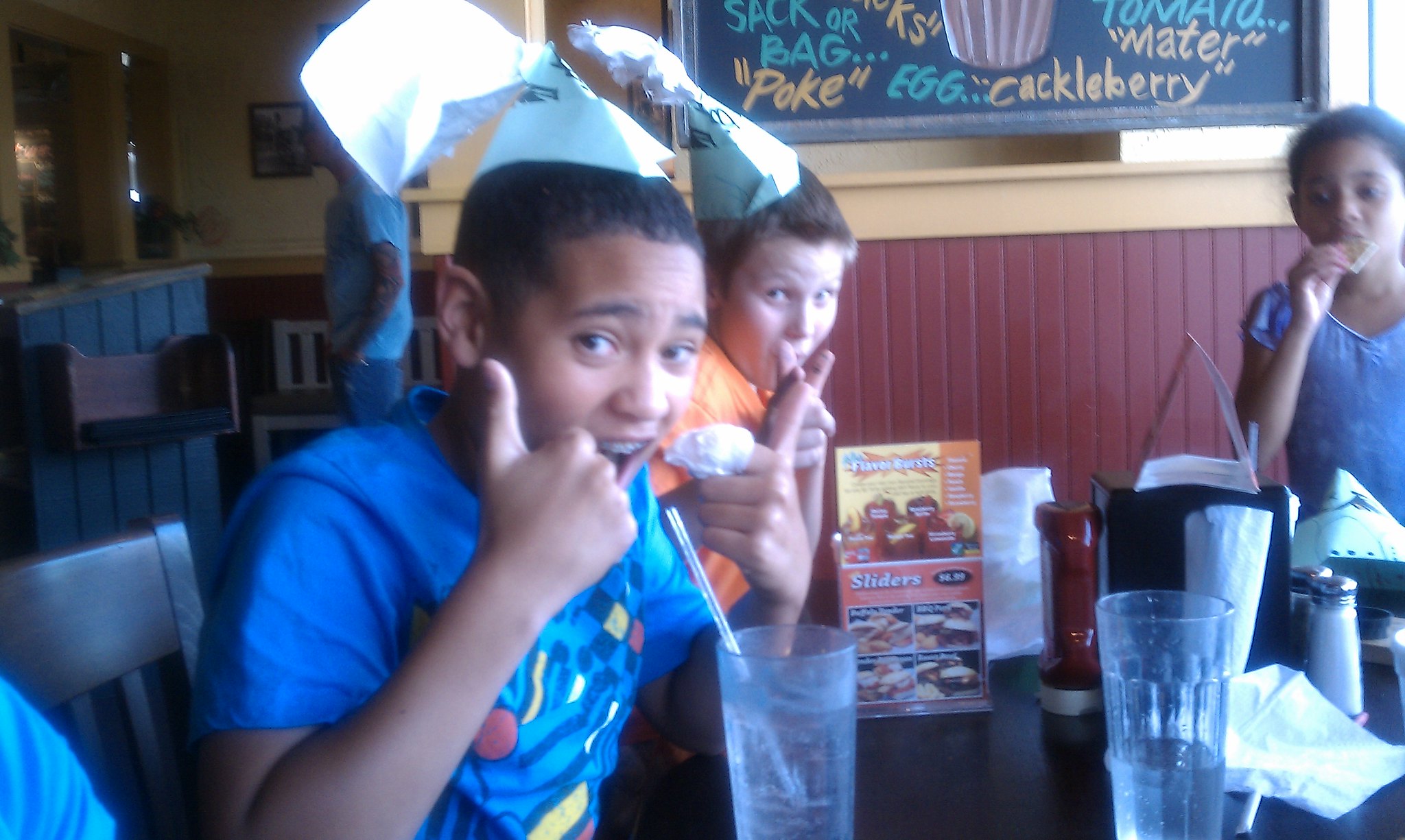In this image, we see three children sitting around a table in a restaurant, captured during what appears to be the middle of the day indoors. The focal point is centered on the kids, who are directly in the middle of the image. The table is cluttered with several objects, including clear glasses, a salt and pepper shaker, napkins, various condiments like ketchup, and a menu. A notable detail on the table is a poster or menu card displaying partially readable text that includes the words "favorite" and "sliders."

The children are wearing paper party hats, adding a festive atmosphere. On the left side, there is a boy with dark skin, black hair, and a blue shirt. He has a napkin twisted around one of his fingers and is giving a thumbs-up with his elbow bent, looking directly at the camera. Next to him, but more in the background, is another boy with light brown hair and a fair complexion, wearing an orange shirt. He too is looking towards the camera. On the right side of the image sits a girl with black hair, wearing a blue dress and eating something that looks like toast or bread. She appears to be around 8 to 10 years old.

Behind the main table, more tables can be seen, along with various posters and decor adorning the walls. The color palette of the scene includes shades of blue, brown, red, yellow, light blue, orange, and gray, contributing to a vibrant and lively atmosphere. Overall, the image captures a cheerful moment among three kids in a colorful and bustling restaurant setting.